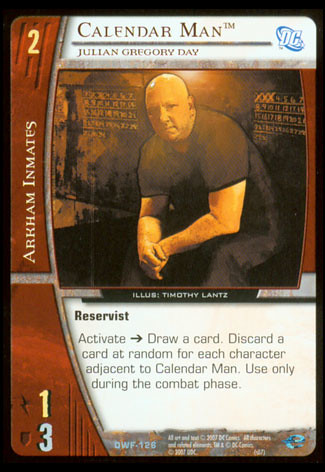This image is a detailed scan of a trading card set against a dark background, featuring a character named "Calendar Man™." The card's focal point is a portrait of a bald, white male, seated and wearing a black t-shirt and black pants, with his hands in his lap. This image is attributed to illustrator Timothy Lance. The man's name is Julian Gregory Day, also known as Calendar Man, and he is depicted against chalkboards with dates and calendars sketched on them, adding to the thematic detail.

In the upper left corner, the card displays the number "2," with vertical text next to it reading "Arkham Inmates." Below this, smaller text reads "Reservist" and "Activate," followed by gameplay instructions: "Draw a card, discard a card at random for each character adjacent to Calendar Man. Use only during the combat phase."

On the right side, there is a prominent DC Comics logo, represented by two royal blue circles containing the letters "DC." The lower section of the card features symbolic game-mechanics elements: a lightning bolt with the number "1" and a shield with the number "3." The footer area of the card also contains additional, though largely unreadable, text likely related to copyright and game-specific information.